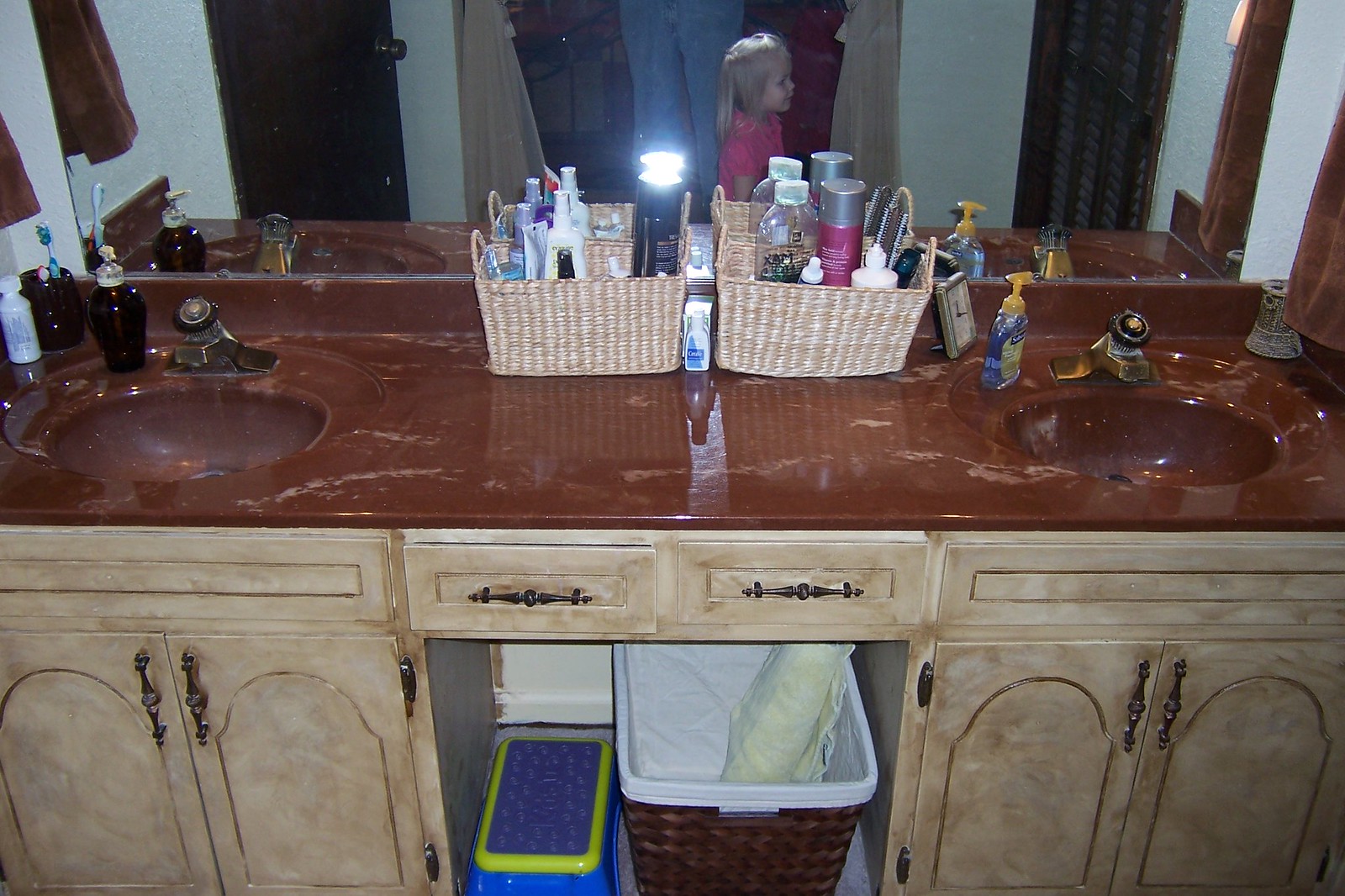The image is of a bathroom with a detailed, reflective scene captured in a large mirror. Centered in the reflection is a brown towel, a toothbrush, and a section of the white wall next to a black door. The window is flanked by curtains in a gradient of blue shades, ranging from light blue to dark blue.

In front of the mirror, a young girl with blonde hair, wearing a pink shirt, is partially visible. Below the mirror and to the upper left, there is a brown marble countertop spanning the sink area. On this countertop, a soap dish and a soap pump are situated next to a toothbrush holder containing the toothbrush.

Beneath the sink, two baskets filled with various items sit on either side. These items include a mix of white and blue objects, one pink item with a gray cap reminiscent of a water bottle, and a small clock near the right basket. Another soap pump sits to the right of the right basket, aligned with the tan marble sink area.

The vanity unit consists of drawers and cabinets with an open space underneath where a trash can is located, holding a white and a yellow item. Adjacent to this is a small blue step ladder with yellow accents. The overall scene is framed by white and gray walls, creating a subtle yet varied color palette in the bathroom decor.